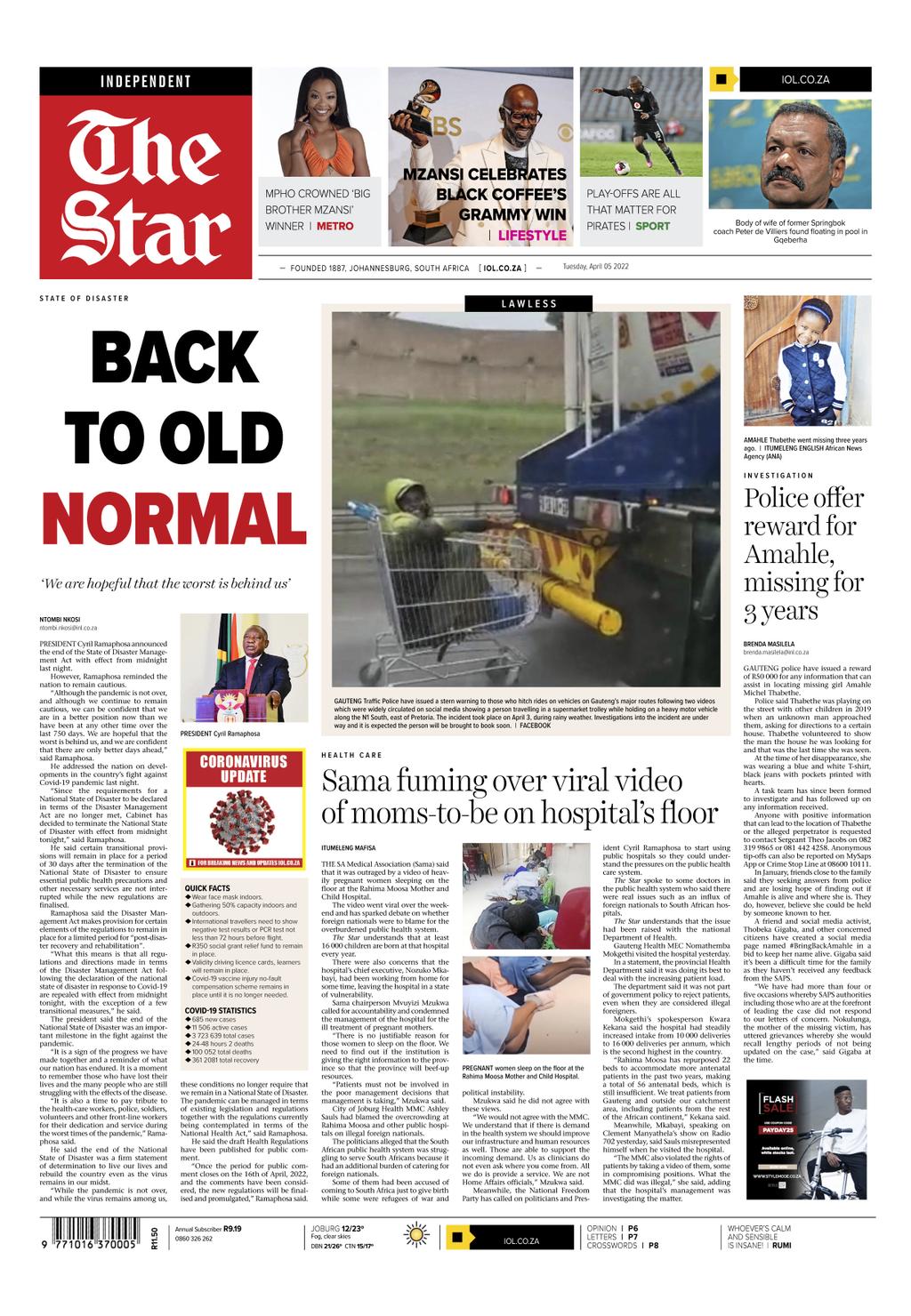The image showcases the layout of the online edition of "The Star" newspaper. On the left-hand side, there's a prominent red box with the bold title "The Star." 

Directly beneath, the first featured article highlights Mpho's recent victory on Big Brother, accompanied by a picture of the woman. 

To the right of this section, another block celebrates Black Coffee's Grammy win.

Following this, an article discusses the importance of playoffs for the Pirates, marked with a related image.

The last block displays a man looking to the left, with some unreadable text beneath him.

At the top of the website, a horizontal bar runs the width of the page, made up of small photos positioned side by side, creating a continuous banner effect.

Finally, the main article, centrally placed below these sections, is titled "Back to Old Normal."